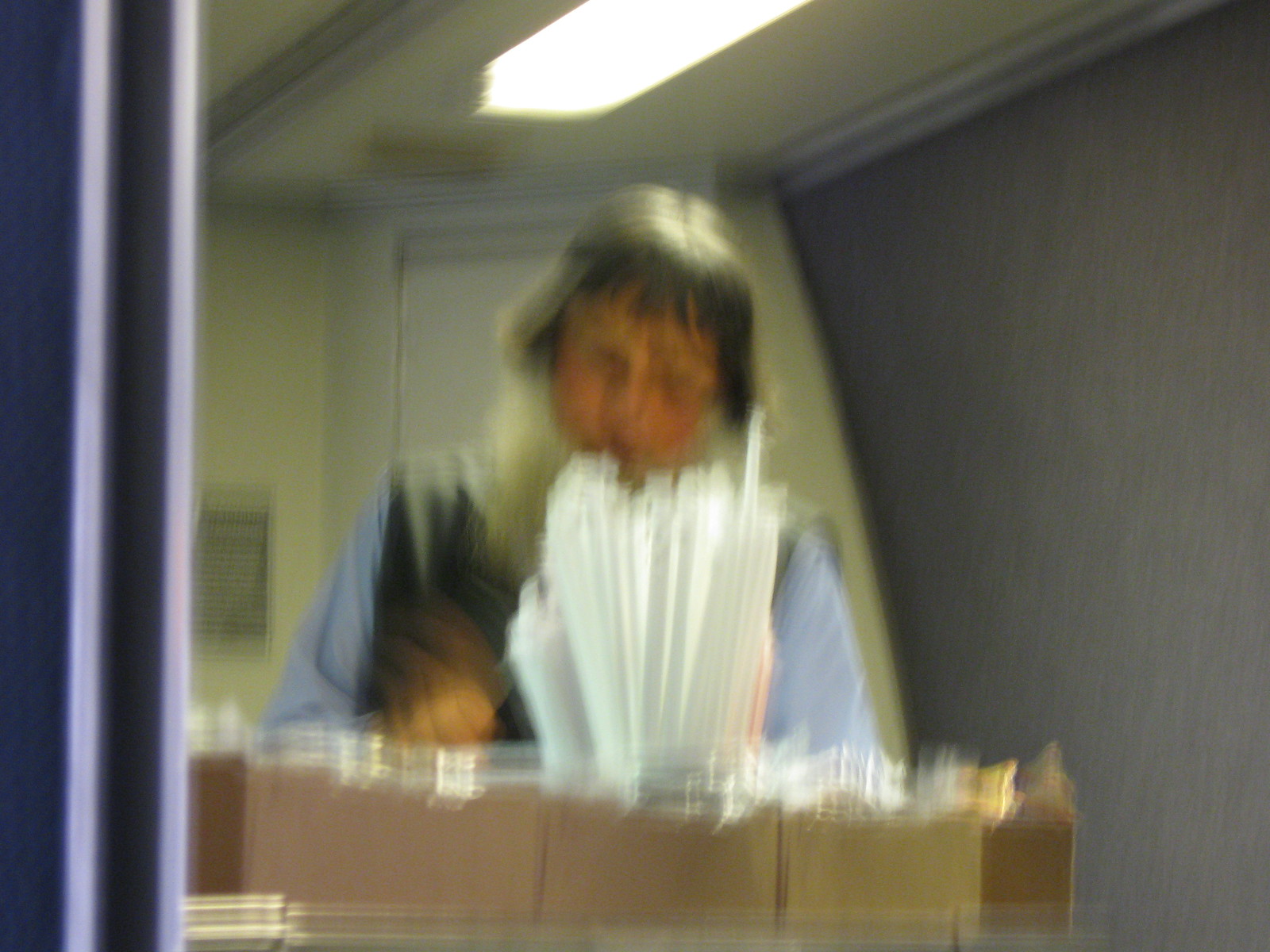This is a color, landscape-format photograph, characterized by significant blurriness, likely due to motion. The image captures a woman, estimated to be between 20 and 40 years old, with short to medium-length brown hair and white skin. She appears to be looking down and concentrating, possibly engaged in writing or examining something. The woman is wearing a long blue shirt, possibly layered under a brown vest, though the details of her clothing are difficult to discern due to the blur.

In front of her are several boxes with uneven tops, containing bunched-up white items that might be straws or pieces of plastic. The photograph suggests she's in an office or indoor setting, discernible by the large fluorescent light fixture above her. To her left, there is a silver or gray plaque on a beige wall, and further left, a couple of purple lines that resemble curtains. The overall scene is contained within a small enclosed space, with some indication of a short door nearby.